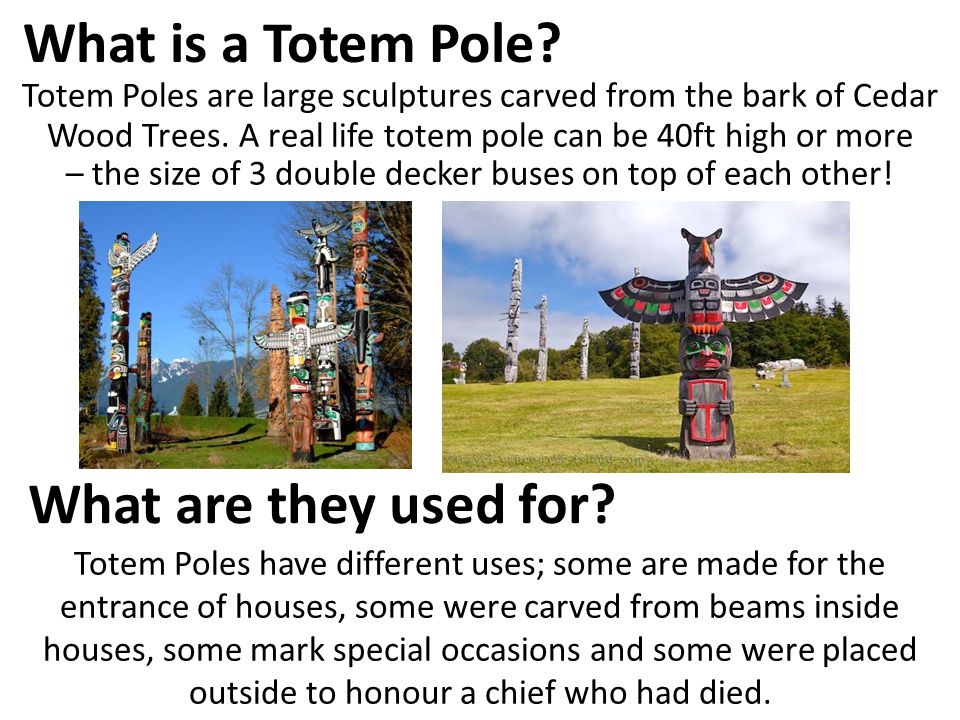The image serves to explain the purpose of totem poles and features black text prominently displayed on a white background. The central part of the image includes two photographs showcasing multiple totem poles. Above these photos, the headline "What is a totem pole?" clearly stands out, followed by explanatory text: "Totem poles are large sculptures carved from the bark of cedar wood trees. A real-life totem pole can be 40 feet high or more, the size of three double-decker buses on top of each other." Below the photos, another headline, "What are they used for?", leads into detailed information: "Totem poles have different uses. Some are made for the entrance of houses. Some were carved from beams inside houses. Some mark special occasions, and some were placed outside to honor a chief who had died."

The first photograph features a group of totem poles standing on green grass, with a backdrop of snow-capped mountains, a big blue sky, and pine trees. These totem poles vary in height, with some adorned with birds on top, their wings spread wide. Faces with beaks, teeth, and intricate designs in greens, yellows, and reds are carved into the poles, alongside one predominantly brown pole with etched designs that are difficult to make out. The second photograph highlights a large totem pole in the foreground, starting with a bird-like figure at the top, complete with a beak and ears, followed by wings and a bird's body clutching a smaller figure's head. Further down, the pole features a face with green around the eyes and red lips, finishing with hands holding a red-outlined shield. The background consists of whitish stone-colored totem poles on a grassy hill, surrounded by trees and set against a cloudy sky.